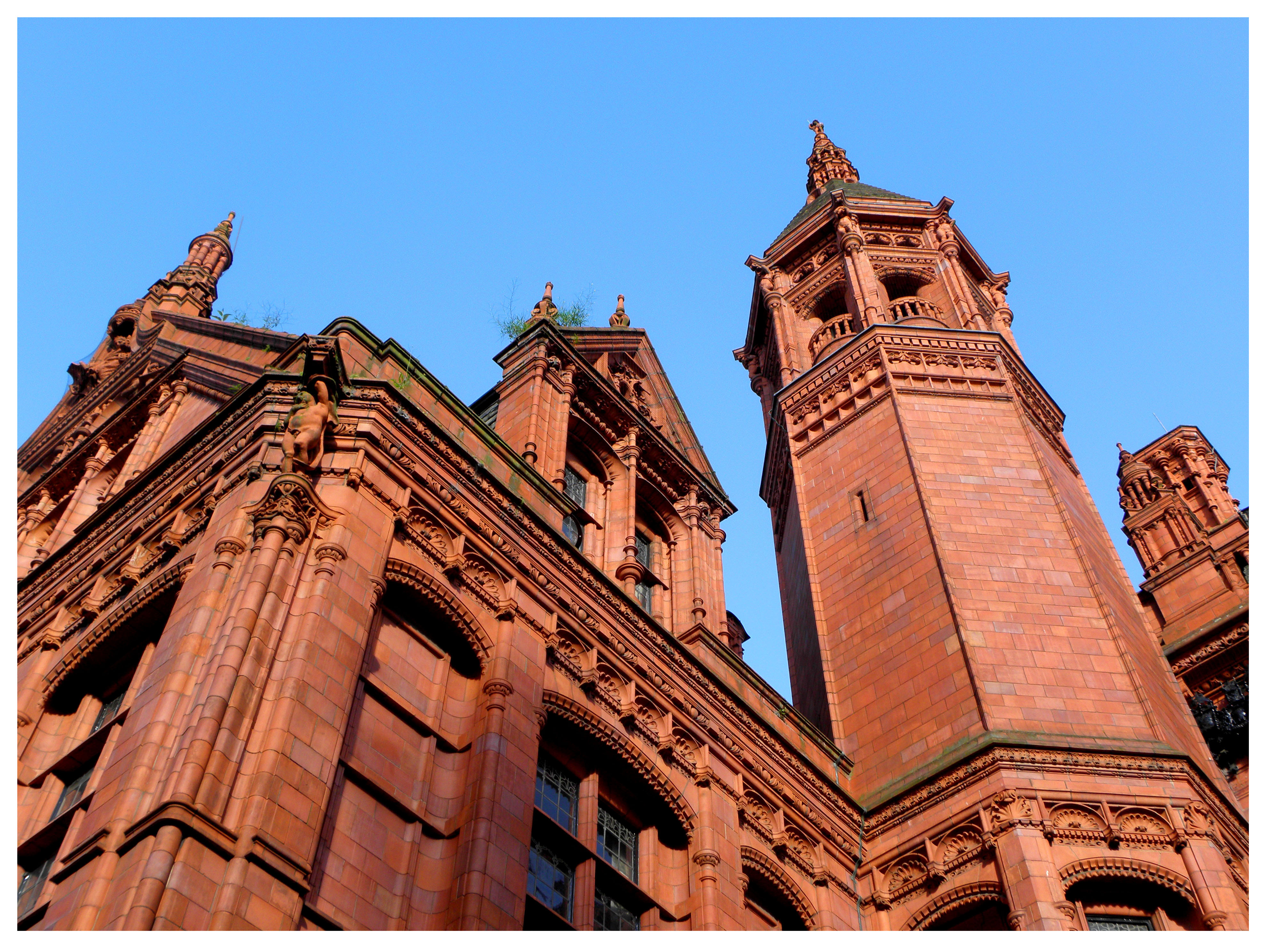In this photograph taken outdoors during a clear, cloudless daytime, we are looking up at an old, well-maintained stone building composed of rectangular blocks in varying shades of orangish-red, interspersed with lighter and darker hues and touches of gray, purple, and blue. The building features a prominent tower on the right-hand side and several arched windows at the base of the tower and across the left side. Atop one corner on the left, there's a statue that appears to be of a person, although the details are indistinct from this angle. The structure is adorned with multiple decorative elements, including turrets and small columns around some windows, along with spirals on the peaks and intricate carvings on the dormers. The top section of the building has repeated rows of decorative embellishments, adding a complex, layered look to the design. There's even some greenery, possibly weeds or moss, growing along the rain gutters. The strikingly brilliant blue sky serves as a backdrop, enhancing the building's impressive and intricate architecture.